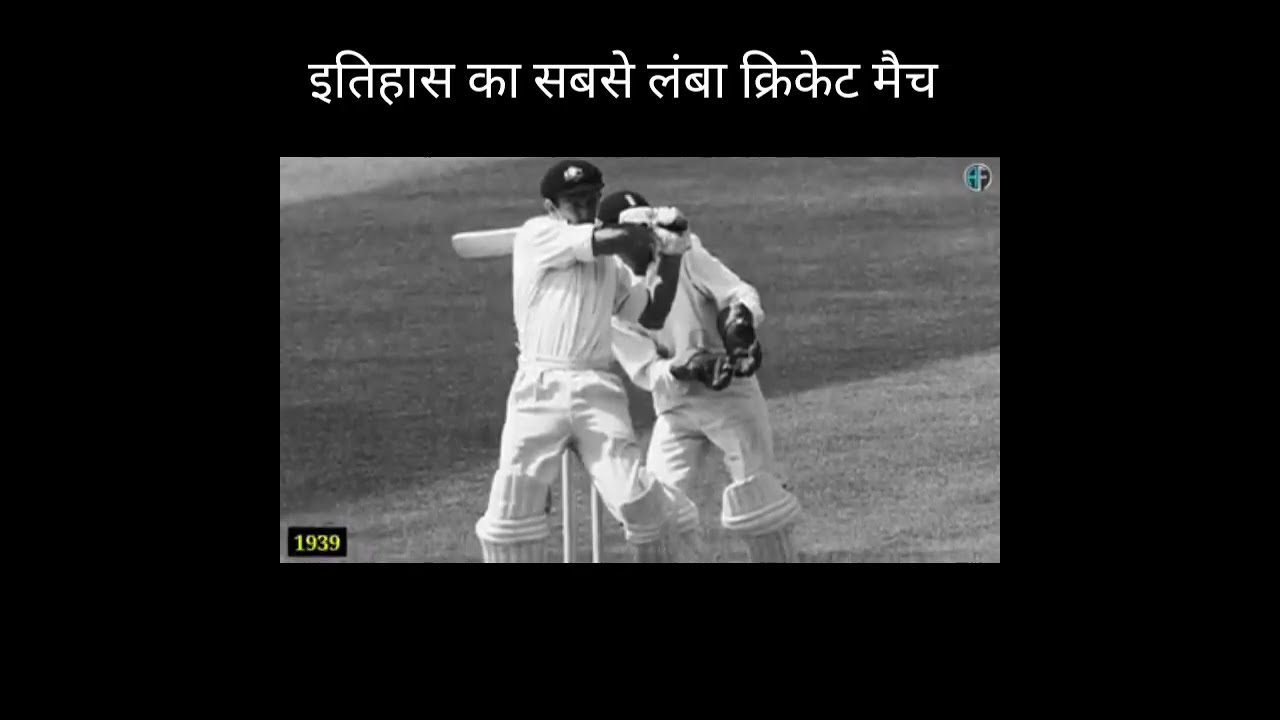The image is a black and white photograph framed by a thick black border. At the top of the frame, there is text in a foreign language, possibly Indian, indicating the prominence of cricket in that region. The primary focus of the photo is two men in white uniforms with black caps and protective knee pads, suggesting they are cricket players. The player on the left appears to have just swung a wide, flat bat or paddle, which is positioned behind his back. Adjacent to him, the second player seems to be leaning back slightly, almost as if avoiding the swing. Both are standing on what appears to be short grass. At the bottom left corner of the image, "1939" is displayed in white text within a small black rectangle, indicating the year the photograph was taken.